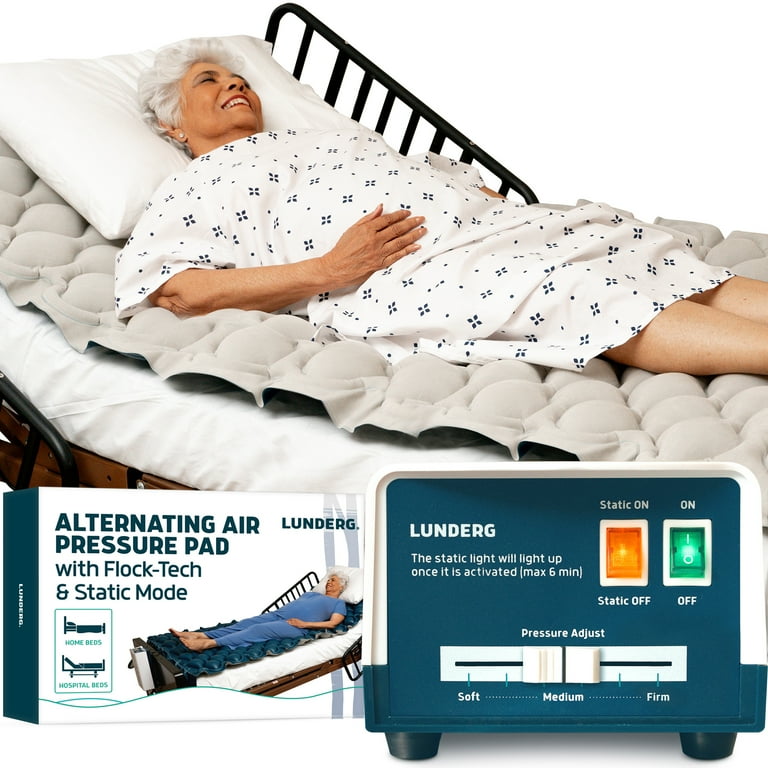This advertisement poster features a photograph of a white-haired woman, possibly a hospital patient, lying contentedly on an adjustable hospital bed with black metallic railings. The bed's head is elevated and is adorned with a white pillow and a gray, bubble-textured comforter. The woman is dressed in a white hospital gown with dark designs and is wearing silver or diamond earrings, bright lipstick, and a noticeable smile with closed eyes.

Below this peaceful scene, the advertisement showcases an air pressure device designed for beds. On the left, the product's packaging displays a blue and white design with various text details, such as "alternating air pressure pad with flop tech and static mode." It also depicts the same woman in different attire lying on both home and hospital beds, with corresponding labels and an image of the blue and brown frame beds.

To the right, the actual device is presented. This machine features a green and white body with distinct buttons and adjustments: an orange "static on/off" switch, a green "on/off" button, and a slider for "pressure adjust" settings marked as soft, medium, and firm. The text on the device reads, "Lunderg, the static light will light up once activated, max 6 min." The product appears to be geared towards enhancing patient comfort through customizable air pressure settings.